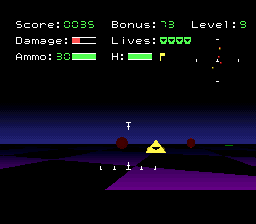A detailed screenshot of an older video game, seemingly from the late 70s or early 80s Atari generation, shows a complex HUD at the top and a mysterious game environment beneath. The HUD displays a score of 35, a bonus of 73, and indicates the player is on level 9. The damage bar reveals that only a small amount of red remains, symbolizing considerable damage taken. The player has 4 lives left, represented by small square icons, and 30 units of ammo, as indicated by a green bar. Another measure labeled "H" is fully green, with a small flag icon next to it. The game environment features a dark checkerboard floor in purple and black, reminiscent of nighttime. The ground is populated with various objects, including red spherical shapes in the distance and a striking yellow triangle resembling a Triforce with an inverted empty space in the middle. The sky is dark blue, transitioning to black, enhancing the overall enigmatic atmosphere of the game.